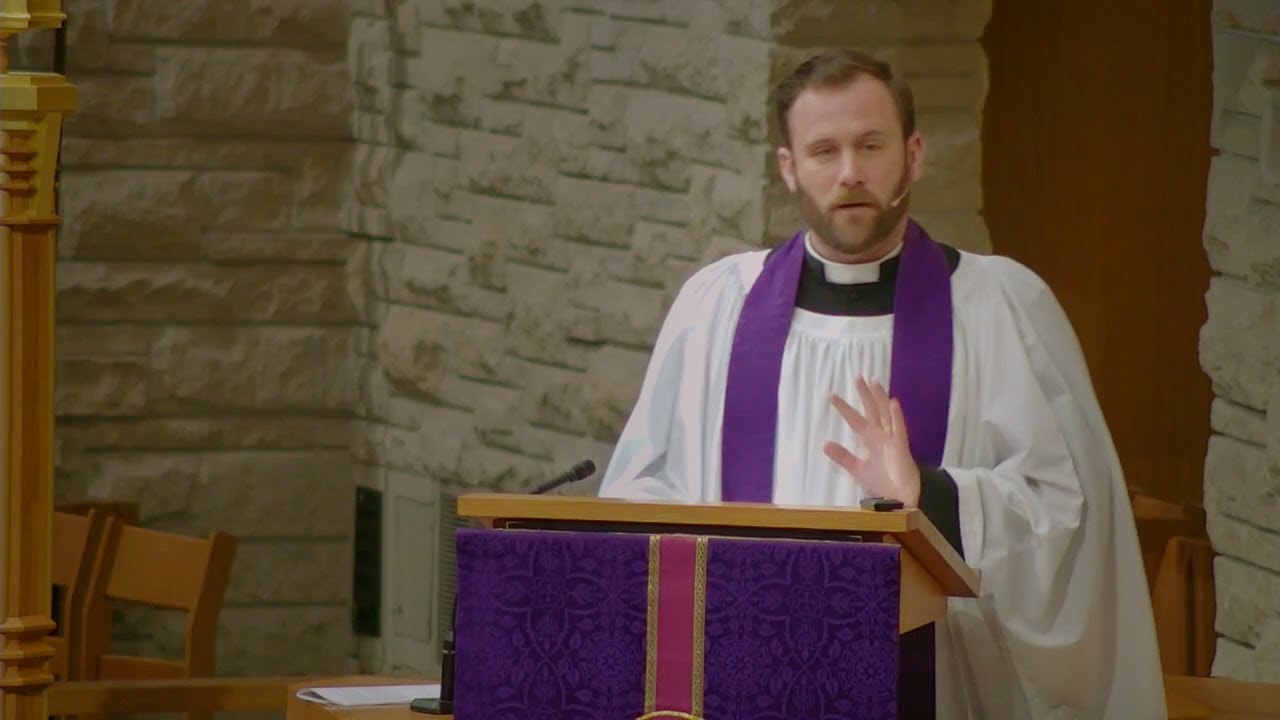This detailed photograph depicts a Caucasian preacher or priest, dressed in traditional vestments, standing at a wooden lectern adorned with a purple, maroon, and gold cloth. His attire includes a black garment layered under a white robe, a distinctive white collar, and a long purple sash draped around his neck. He has a close-trimmed brunette beard and wears a microphone on one ear, complementing another small microphone situated at the front of the lectern. The stone walls of the church form the backdrop, with a wooden pillar, parts of chairs, and other indistinct furniture visible on the periphery. The scene conveys an image of the preacher delivering a sermon or addressing an audience.